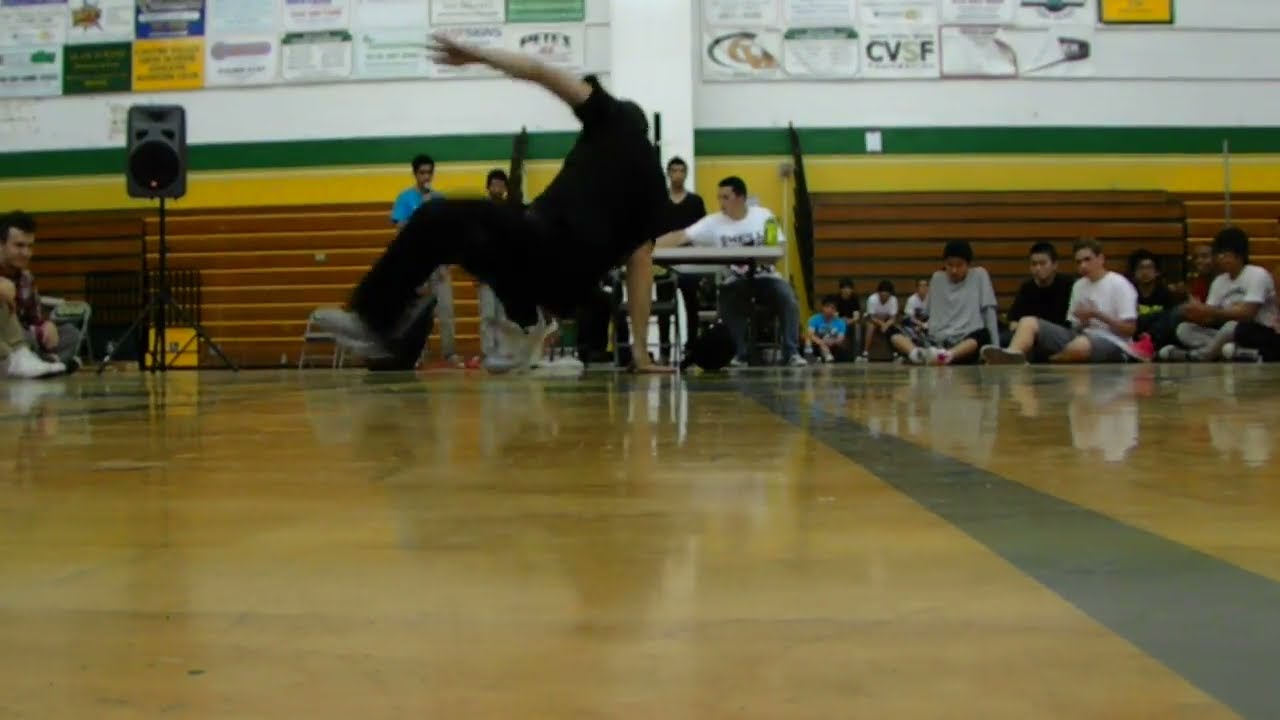The image is a horizontal rectangular photograph taken inside a school gymnasium. The backdrop features a wall with a lower section of brick, followed by a broad yellow stripe, and a slightly narrower green stripe above it. The upper part of the wall is adorned with numerous rectangular posters, advertisements, or announcements, though the details on them are not legible.

In the foreground, the polished wooden gym floor gleams, typical of a basketball court. The camera angle is low, offering an exaggerated close-up of the shiny floor. On the right side, there's a broad stripe marking the court.

At the center of the image, against the wall, is a plastic folding table where three young teenagers are positioned: two sitting behind the table on metal folding chairs and one standing behind them in a black sweatshirt. The table holds two trophies, suggesting a competitive event. In front of the table, there appears to be someone breakdancing; the body is in a twisted pose with motion blur, making details slightly unclear. This central activity catches the attention of several young boys sitting cross-legged on the floor to the right, all dressed in shorts and t-shirts, likely spectators. 

On the left side of the table, two individuals in blue t-shirts stand, one of them holding a microphone, near a large speaker box. Further left, a small group of people are standing near the wall, adding to the bustling environment. The entire scene is dynamic, filled with energy and anticipation, centered around the performance or competition taking place on the gym floor.